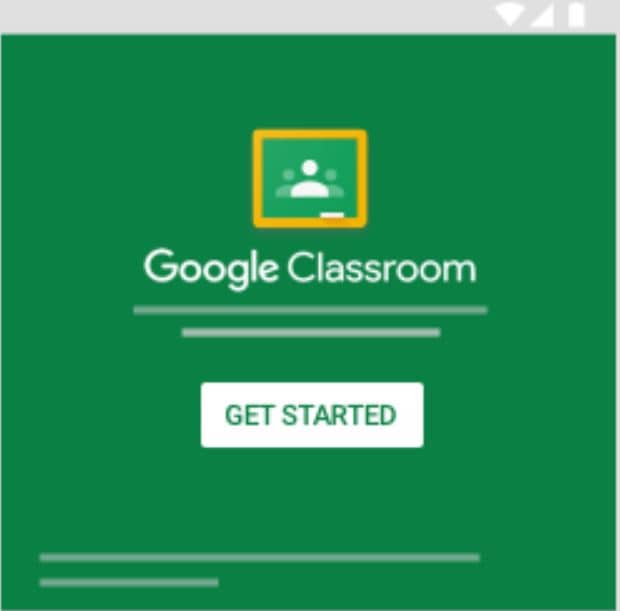The screenshot from Google Classroom features a clean and organized interface. At the top, a thin gray rectangle spans the width of the screen. In the upper right corner, three status icons indicate Wi-Fi connectivity, service status, and battery life. 

The main section of the screenshot presents a green background, centrally showcasing the Google Classroom logo, which consists of a yellow square outline filled with a lighter green. Within this logo, three illustrated figures are depicted, symbolizing a group or classroom. 

Positioned near the bottom of the logo is a small white rectangle resembling a piece of chalk. Directly below the logo, "Google Classroom" is written in a clean, readable font. Underneath this text are two horizontal gray lines; the first line is longer and the second one beneath it is shorter. 

Further down, a prominent white rectangular button with green text urges the user to "Get Started." At the very bottom of the screenshot, two additional gray lines are visible: the first line being the longest on the page and aligning across the screen, while the second, shorter gray line is offset to the left below it.